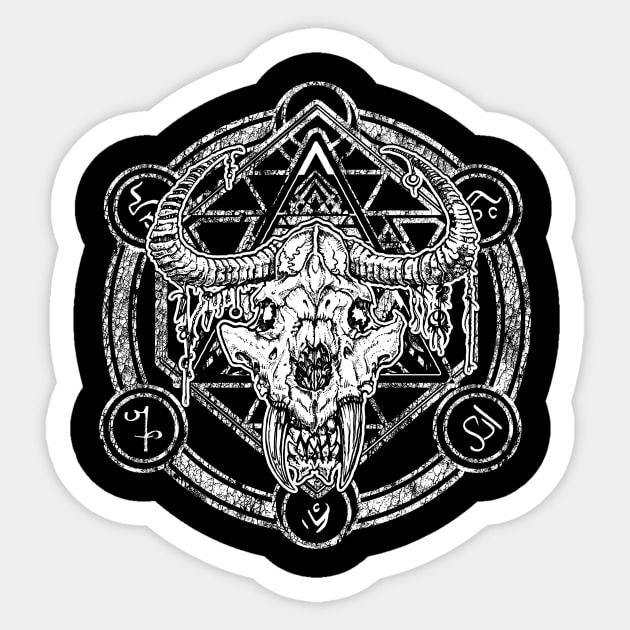This image is a detailed black-and-white product photograph of what appears to be either a sticker or an iron-on patch. It features a highly intricate and monstrous skull at its center, which looks to be a blend between a feline, goat, or cow, bearing enormous fangs protruding from its mouth. The skull sports a pair of curved horns adorned with various ornate items dangling from them, and its starry eyes add to its mysterious allure. Surrounding the skull is an array of occult and runic symbology embedded within multiple circles that encompass the central figure. Additionally, there is a hexagonal geometric pattern framing the skull, with a prominent pyramid and chevron positioned above its head. The entire design is meticulously rendered and exudes a dark, almost satanic aesthetic.